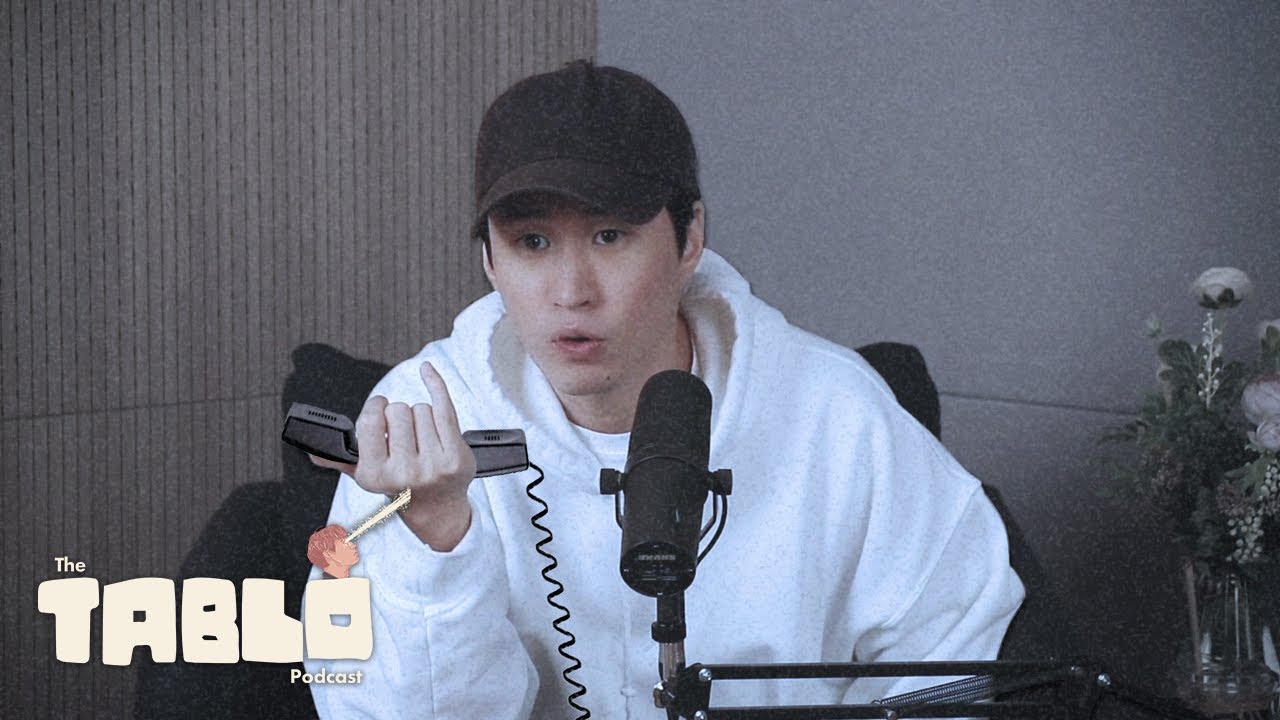In this digitally edited medium shot, an Asian man in his late 20s or early 30s is the focal point. He has black hair, dark brown eyes, and black eyebrows. He is wearing a black baseball cap, a white hoodie, and a white t-shirt. The man is sitting in a dark-colored chair holding a phone handset in his right hand with his pinky finger raised, appearing mid-speech. In front of him is a black microphone, and to his left is a clear vase containing white flowers and green foliage. The background features two distinct walls: one with gray paneling on the right and another with light brown wooden slats on the left. The lower third of the image displays the words "The Tableau Podcast," with a pink plunger-like object above the "O" in "Tableau."